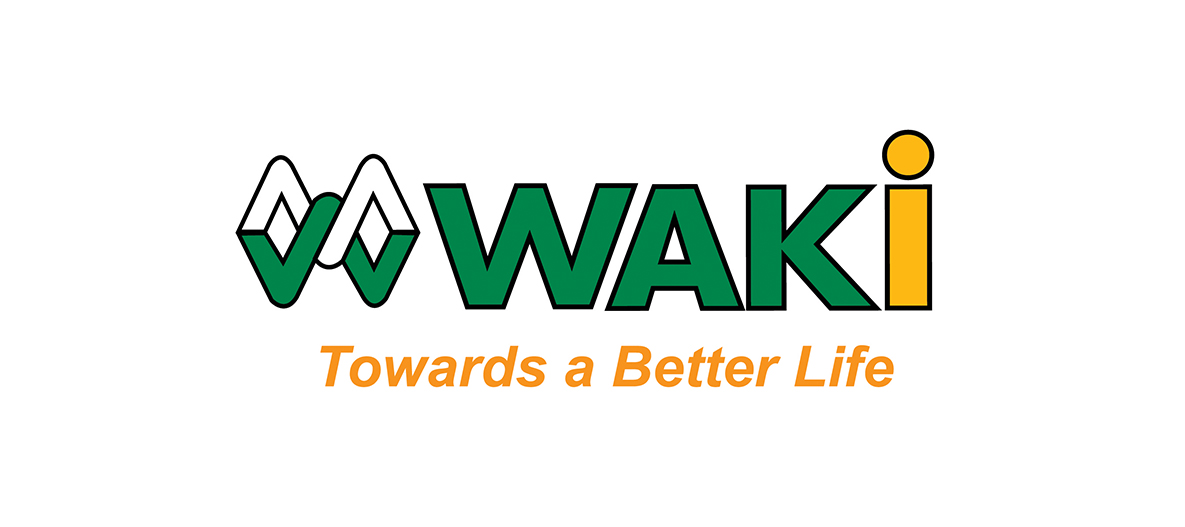The image features a logo set against a white background. At the center top, the logo prominently displays the word "Wacky" in all capital letters. The letters 'W,' 'A,' and 'K' are green with a thin black outline, while the letter 'I' is yellow with a black outline and a yellow dot. To the left of the word "Wacky," there is an insignia that resembles a twisted square or a combination of the letters 'M' and 'W' stacked together. This emblem is colored in white and green with black framing. Below "Wacky," in a much smaller, plain orange font without an outline, the phrase "Towards a Better Life" is inscribed, suggesting the company's aspirational mission.